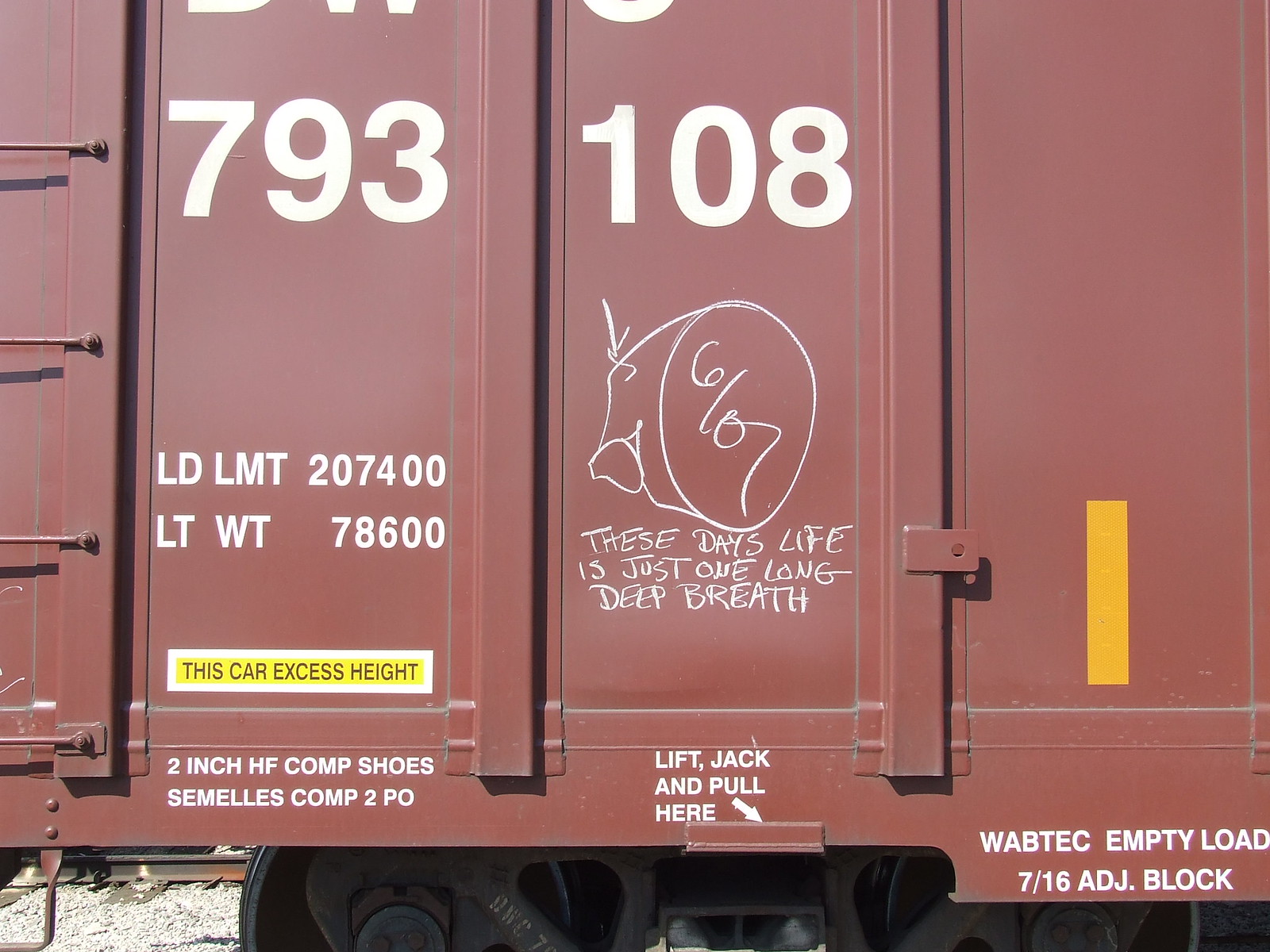This image is a close-up photograph of a section of a cargo train car, painted in a dark terracotta or reddish-brown color. Prominently displayed in large white numbers are "793108" on the side of the car. The car features several vertical reinforcing bars spread evenly along its length and a metal ladder leading upward. Various operational texts are visible, including "this car excess height," "lift jack and pull here," "LD LMT 207 400," "LT WT 78 600," and "empty load 7/16th ADJ block." Notable at the center of the car is a piece of graffiti with the phrase, "these days life is just one long deep breath," accompanied by a drawing with the numbers "6/07." The ground below is pale gravel, and a glimpse of the train's wheels is visible beneath the car. Additionally, a yellow sticker emphasizing the car's excess height is affixed to the right panel.